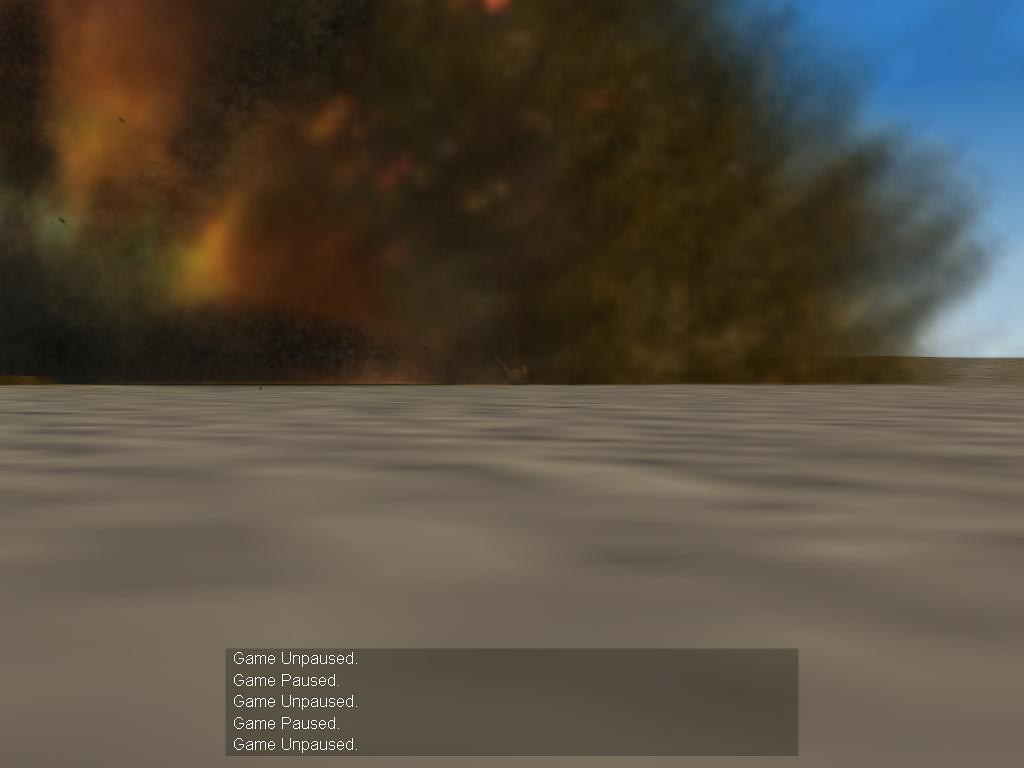The video game screen showcases a dynamic and visually striking scene. The bottom half of the screen is dominated by an expansive spread of gray sand, characterized by a rippled texture that adds a sense of movement and depth. Above the sandy expanse, a dramatic event seems to be unfolding. On the left side of the screen, a dark mass suggests an explosion or some form of intense activity. This mass extends upward and diagonally to the right, trailing what appear to be flames and debris in its wake. The sky beyond this tumultuous scene is a clear, calm blue, providing a stark contrast to the chaos below. In the very bottom center of the screen, a small block repeatedly displays the messages "Game Unpaused," "Game Paused," and "Game Unpaused," indicating possible interruptions in the gameplay.